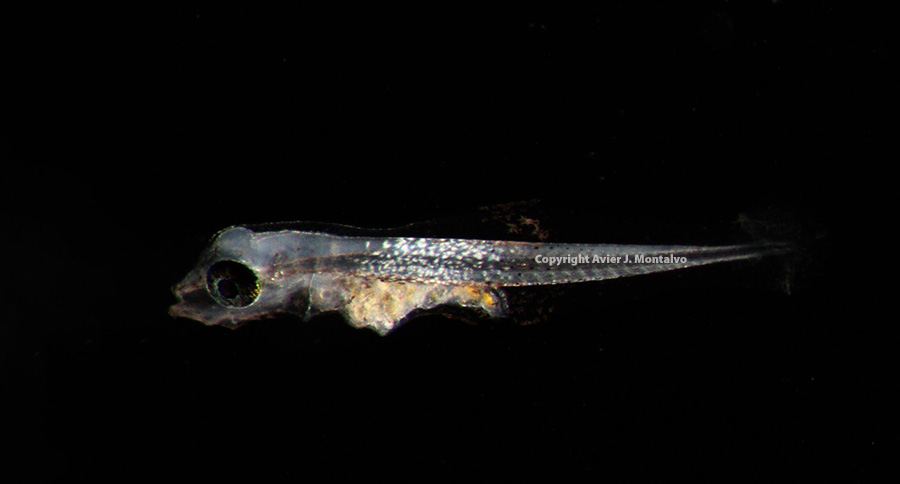This image captures a close-up of a small, possibly freshwater, sea creature set against a pitch-black background. The subject appears semi-transparent, allowing the internal structures to be partially visible, including a prominent black line running through its body. Notably, there is a small, fin-like appendage protruding from its side. The creature features a large, round eye which gives the impression of an empty eye socket due to its translucence. Additionally, inscribed in white text on the creature's body is a copyright notice followed by a name, indicating the photographer or creator's ownership of the image. The detailed and eerie appearance of this mysterious fish provides a fascinating glimpse into the lesser-known inhabitants of aquatic environments.